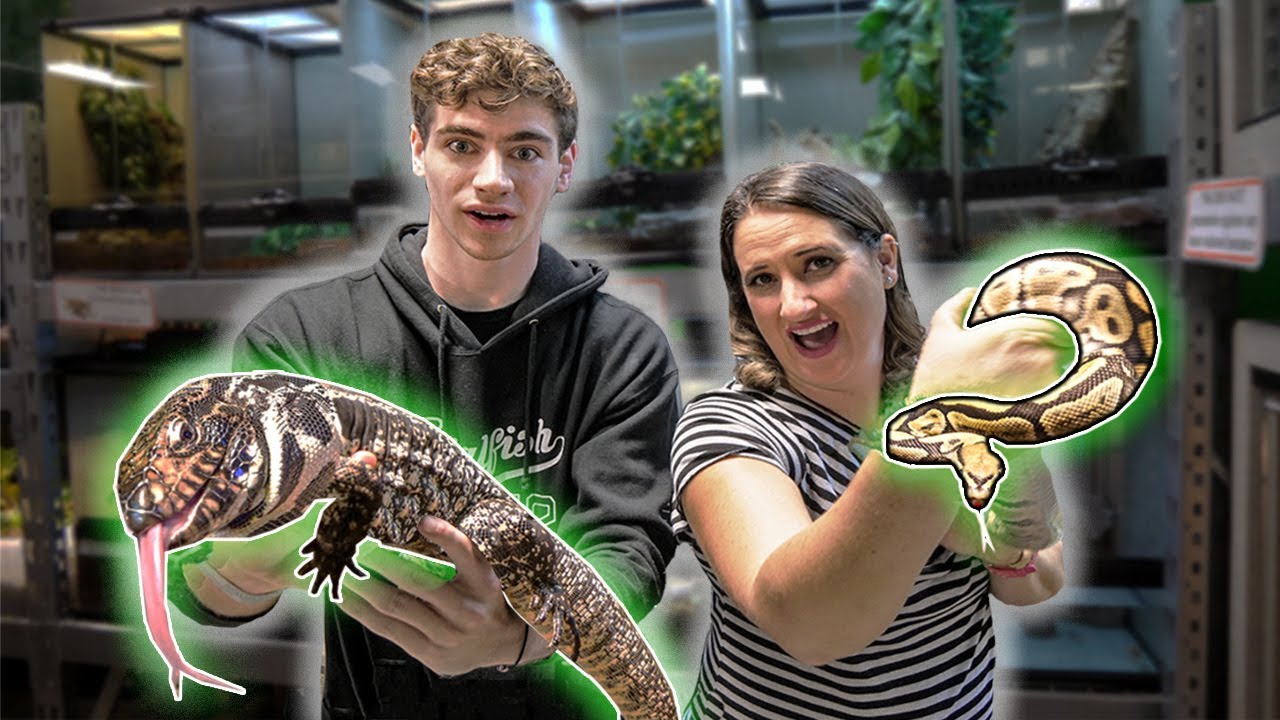In the image, we see a man and a woman, each holding a reptile. The man on the left, dressed in a black hoodie with curly brown hair, has a surprised expression on his face as he holds a large lizard. The lizard, highlighted with a white and green outline, has a striking black, brown, and orange pattern with its tongue sticking out. On the right, the woman, wearing a short-sleeve black and white striped shirt, mirrors the man's surprised expression while holding a snake. The snake, potentially a python, has a spotted pattern in shades of tan, yellow, and brown, and also has its tongue out. The background features blurred aquariums filled with plants, suggesting that they are in a place dedicated to reptiles, such as a pet store or a reptile nursery, possibly for a YouTube video thumbnail highlighting this unique location.